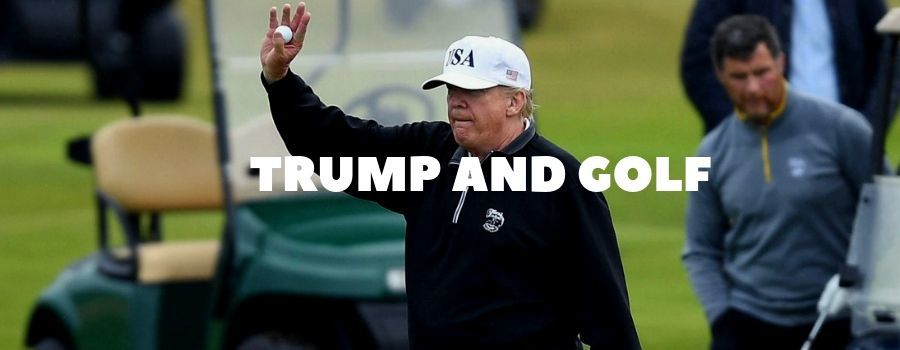In this photograph, President Donald Trump stands at the center, waist up, against a backdrop of a green golf course. Dressed in a black, long-sleeve, half-zip shirt with a gray collar, he sports a white cap that prominently features "USA" in black letters and an American flag on the side. Trump holds up a golf ball in his right hand, appearing to wave at someone off-camera to his left. Behind him to the right, partially visible, is a green golf cart; another golf cart and figures populate the background. One man with black hair, seated on the right, wears a gray long-sleeve shirt with a yellow zipper, while another person, seen from the torso down, is dressed in a blue long-sleeve shirt with a light blue undershirt and holds a golf club. Dominating the middle of the image in large, caps-locked, white text is the phrase "TRUMP AND GOLF".